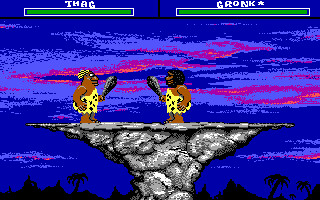In this video game scene, the screen showcases a vibrant royal blue sky adorned with fluffy light blue and soft pink clouds, creating a whimsical atmosphere. The ground in the background features lush palm trees and rolling hills, adding a touch of natural beauty to the setting. Foregrounded prominently is a high stone pedestal, upon which two cavemen stand facing each other, ready for combat with clubs gripped in one hand each. One of the characters is bald, while the other sports a full head of dark hair along with a beard and mustache. Both characters are clad in primitive clothing reminiscent of Tarzan, made from animal skins. Above the bald opponent, the name "Thag" is displayed in white letters, while the other opponent is labeled "Gronk." The scene merges prehistoric elements with an engaging confrontation, setting the stage for an epic showdown.